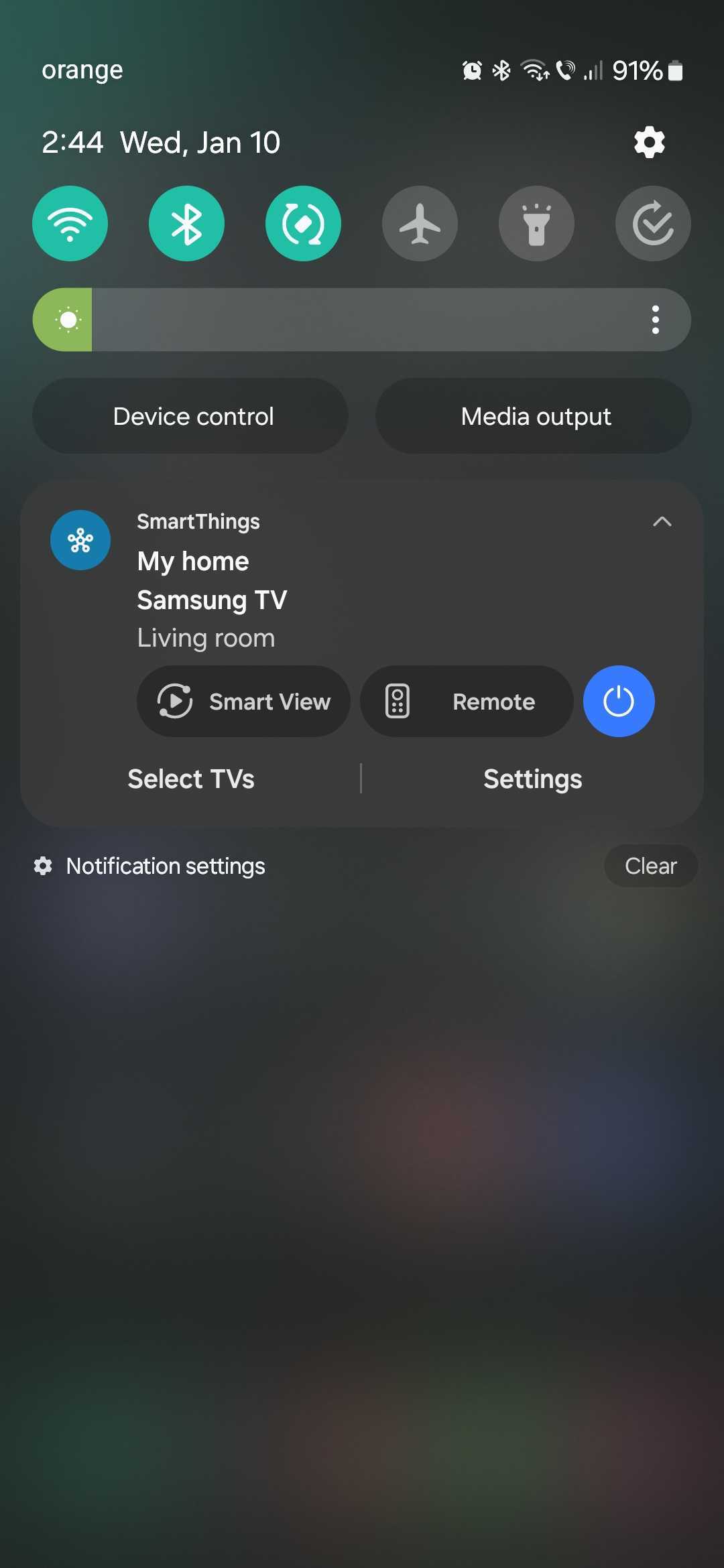This screenshot captures the interface of a smartphone, displaying various status icons and settings. At the top of the screen, there's an orange notification bar that includes essential indicators such as the clock, Bluetooth status, Wi-Fi signal, network bars, and battery percentage, which is at 91%. Directly beneath this bar, the time reads 2:44, although the period (a.m./p.m.) is not specified. The date is noted as Wednesday, January 10th.

Immediately below the date and time, there are toggle buttons for Wi-Fi, Bluetooth, and location services, all of which are currently turned off. Airplane mode is indicated but also turned off, along with the flashlight. There's an additional icon whose function is not identified. The brightness slider is set to a low level.

Further down, there are sections for media control and output. The "Media" section indicates "Device Control" and "Media Output." Below these options is a segment labeled "SmartThings My Home," which lists a Samsung TV located in the living room. Options within this section include "Smart View," "Remote," and "Select TV's Settings," along with a power button suggesting control over a smart TV.

Finally, the screen displays the options "Notifications" and "Settings," alongside a "Clear" button. The rest of the screen below these options is blank, indicating there are no additional items or information present.